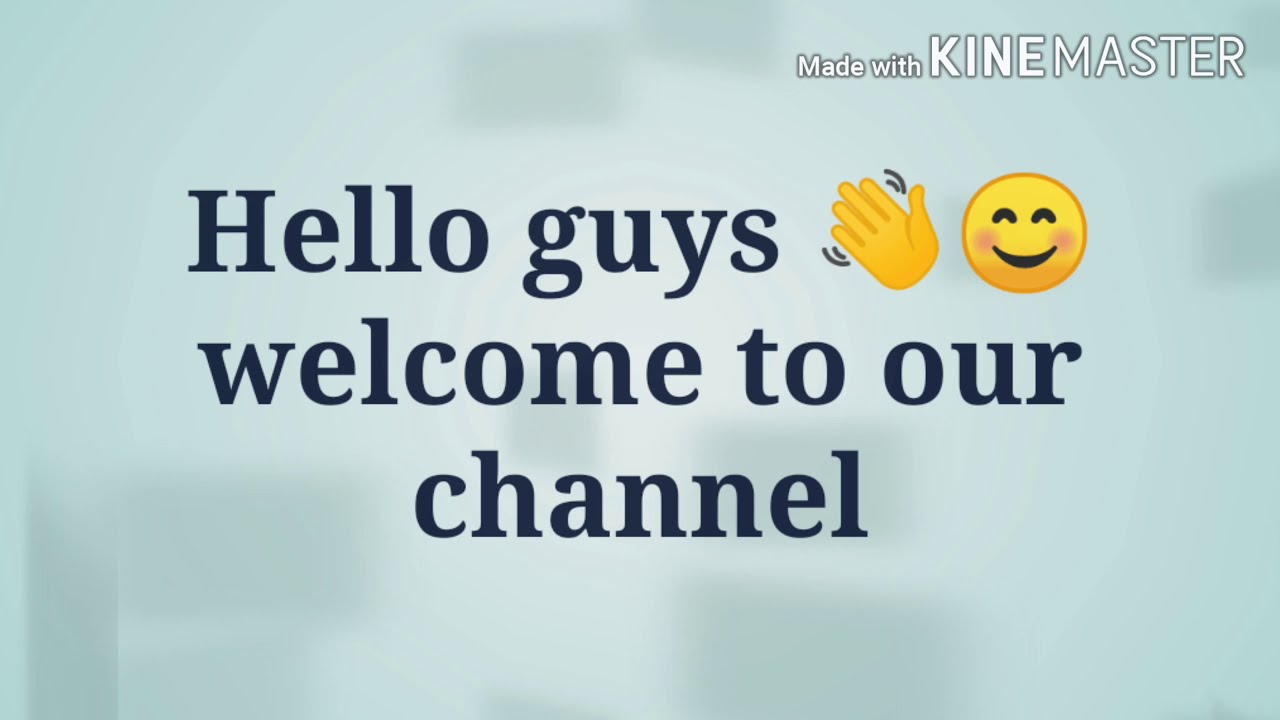This image displays an introductory screen likely used for a YouTube channel, created with the KineMaster app. The top right corner features a watermark reading "Made with KineMaster" in bold, capitalized white letters with "Kine" emphasized. The central text, written in a dark, serif font, reads, "Hello guys, welcome to our channel." Accompanying this text are two emojis: a golden waving hand with gray motion lines and a smiling yellow face with rosy pink cheeks. The background is a muted, light moss green or aqua foamy green, adorned with blurry gray squares of varying sizes, lending a subtle, textured effect. This welcoming screen suggests the start of a video aimed at greeting viewers to the channel.